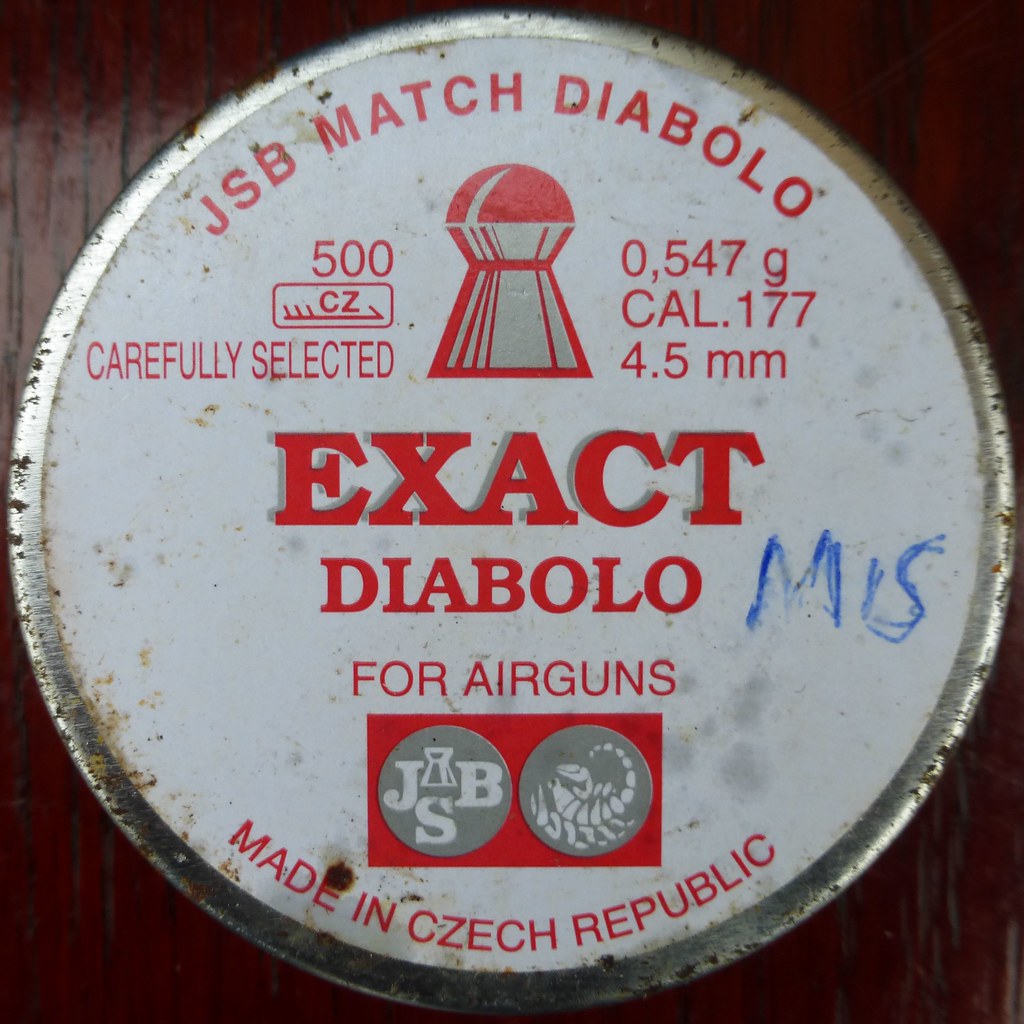This large, square image features a dark brown, cherry-colored wooden surface with prominent vertical black wood grains. On top of this surface lies a large, circular metal object with a rusted silver border featuring brown spots. The face of the circle is white, and at the top, curved in red capital letters, it says "JSB MATCH DIABOLO." 

Beneath this heading, there is a logo resembling a water tower, flanked by the number "500" on the left and "0.547G" on the right. Below this, it states "CAL. 177" and "4.5MM." Prominently in the center, large bold red letters spell out "EXACT," with a smaller "DIABOLO" underneath. On the right side of the word "DIABOLO," there's handwritten text that reads "M.S."

Centered at the bottom of the circle, it declares "4 AIR GUNS." Below this, there's a red rectangular box containing two gray and white circular logos, one of which includes the letters "JSB." Finally, curving along the bottom of the circle, it reads "MADE IN CZECH REPUBLIC" in red capital letters.